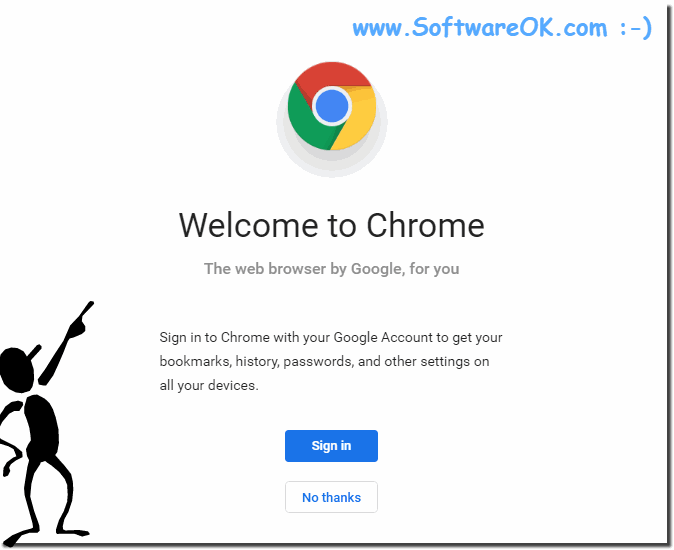At the top right corner of the image, the website URL "www.softwareok.com" is displayed in blue text. To the right of this URL, there is an emoticon made with a colon, a dash, and a closed parenthesis. Below this, on the left side of the image, there is a Windows icon depicted as a circle subdivided into red, yellow, green, and blue quadrants.

In the main section of the image, a message reads: "Welcome to Chrome, the web browser brought by Google for you. Sign in to Chrome with your Google account to get your bookmarks, history, passwords, and other settings on all your devices." Underneath this message, there are two buttons. The first is a blue button with white text that says "Sign in." Below it, there is a white button outlined in gray with blue text that reads "No thanks."

Along the right edge of the image and extending to the bottom edge is a thin line. At the bottom left side, touching the line with his toe, is a stylized black silhouette of a man. This figure resembles a stick figure but with a bean-shaped body and a separate circular head. He has an exaggeratedly long nose, almost as long as his pointing finger, and elongated, stick-like legs and arms. He is pointing upwards towards the Google logo. The entire background of the image is white.